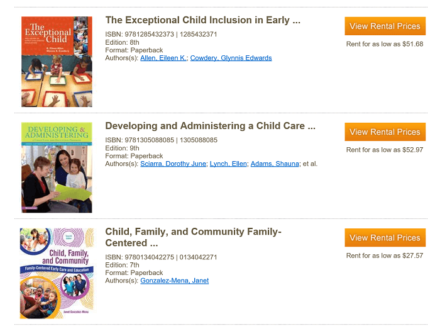This cropped screenshot, taken from an online college bookstore, features a clean, white background and a layout showing three book listings aligned on the left side. Each listing begins with a thumbnail image of the book cover, followed by an orange "View Rental Prices" button on the far right, under which it indicates rental prices starting as low as $51.08. The book titles are listed to the right of each thumbnail, along with additional details underneath including the ISBN number, the editor, format information, and hyperlinked author names in blue. Thin gray lines separate each listing for clarity.

The titles shown in the screenshot are as follows:

1. "The Exceptional Child: Inclusion and Early..." (Title truncated)
2. "Developing and Administrating a Child Care..." (Title truncated)
3. "Child, Family, and Community: Family Centered..." (Title truncated)